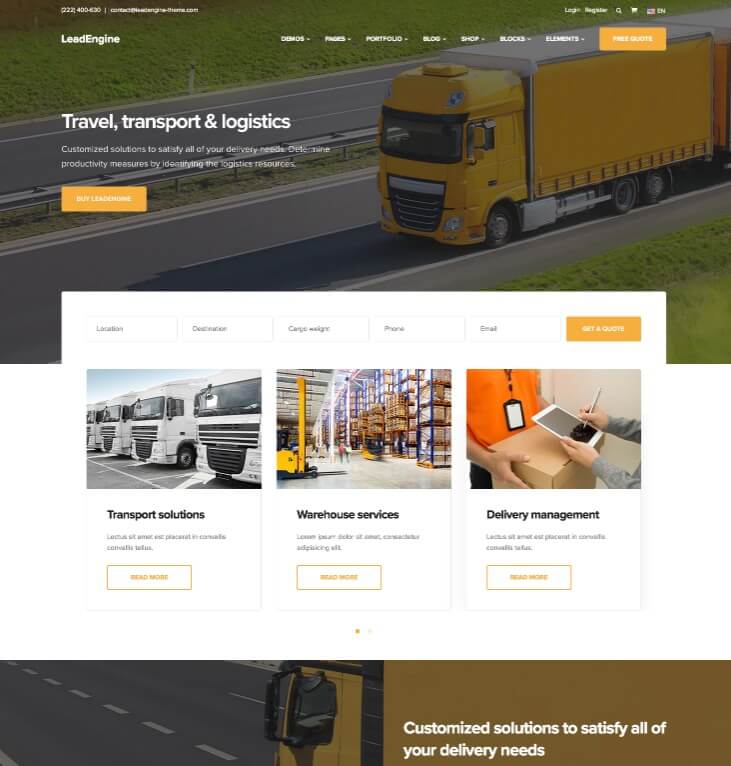The screenshot displays a website for "Lead Engine," which specializes in travel, transport, and logistics solutions. The site emphasizes its capability to customize solutions tailored to meet diverse delivery needs and to enhance productivity by identifying key logistics resources. The branding also references "Lead Line" or "Lead Engine."

At the top of the webpage, there's a navigation bar with dropdown menus labeled: Demos, Prices, Portfolio, Blog, Shop, Blocks, Elements, and a prominent button for a "Free Quote." 

Further down the page, a series of clickable rectangles provide options for "Location" (although one is too blurry to read), "Cargo Worker," "Phone," "Email," and "Get a Quote."

Below this section, additional clickable rectangles present service categories like "Transport Solutions," "Warehouse Services," and "Delivery Management," each positioned side by side.

At the bottom of the screenshot, there is an image of a roadway and a truck within a rectangle, reiterating the message: "Customized solutions to satisfy all of your delivery needs." This text is displayed in white font on a black background.

A yellow semi-truck is visible at the very top of the image, moving towards the left.